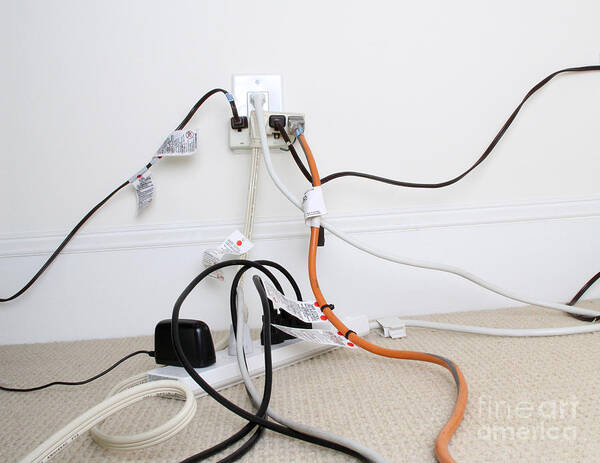In the image, a cluttered array of electrical cords emanates from a two-port wall outlet, indicating a hazardous situation. The top port has a surge protector overloaded with numerous cords in orange, white, black, and a milky off-white hue. The cords are sprawled haphazardly across a light beige patterned carpet, which lies against a white wall complemented by white molding at the base. The surge protector hosts around twelve different connections, with wires jutting out in every direction, suggesting a significant risk of electrical mishap. To top it off, there is a translucent logo reading "Fine Art America" at the bottom of the image, underscoring the dire need for urgent intervention to prevent potential danger.